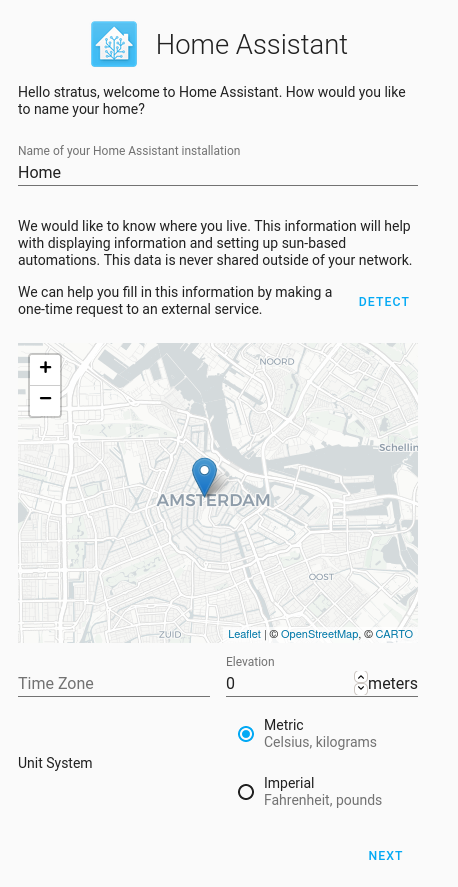This is a detailed screenshot taken from a smartphone screen, specifically showcasing the initial setup interface for the Home Assistant application. 

At the top left corner of the screen, there is a blue rectangular box featuring a white house icon adorned with blue vine-like embellishments that blend with the background. To the right of this icon, centralized but more towards the left, is the title "Home Assistant."

Beneath the title, a friendly greeting, "Hello Stratus, Welcome to Home Assistant," is displayed, followed by a prompt asking, "How would you like to name your home?" The text field below asks for the "Name of your Home Assistant Installation," and a default suggestion "Home" is visible on the left side, separated by a black line.

Further down, the interface requests, "We would like to know where you live. This information will help you with displaying information and setting up Sun-based automations. This data is never shared outside of your network." It then offers assistance in filling out this information with a one-time request to an external service, indicated by the word “Detect” positioned to the right.

The screen displays a map of Amsterdam marked with a location pin. Underneath the map, the location-specific settings such as "Time Zone," with "Elevation 0" to the right, are laid out. Measurement units are selectable with "Metric" highlighted within a blue circle, followed by "Imperial."

Finally, at the bottom right, the interface provides a "Next" button for proceeding with the setup process.